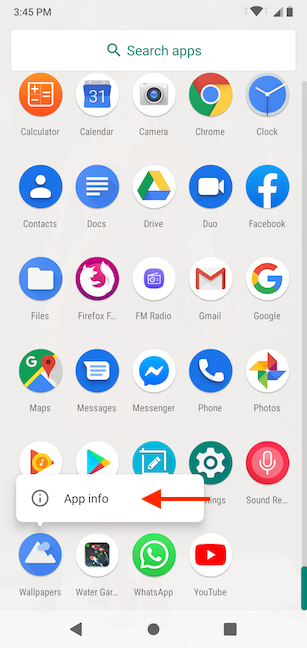The image is a vertical screenshot, resembling the aspect ratio typically displayed on a smartphone such as an iPhone or an Android device. The background is entirely gray. In the top-left corner, "3:45 PM" is displayed in black text, indicating the current time. The top-right corner shows a Wi-Fi icon with three out of four bars filled, and a fully charged battery icon just beside it.

Beneath this, there is a long, rectangular white search bar with a blue magnifying glass icon on the left and the text "Search apps" in blue letters in the center. 

Below the search bar, there are six rows of app icons. Each icon has its name displayed in gray text underneath it. The layout is as follows:

- **First Row (Left to Right):** Calculator, Calendar, Camera, Chrome, Clock.
- **Second Row (Left to Right):** Contacts, Docs, Drive, Duo, Facebook.
- **Third Row (Left to Right):** Files, Firefox, an 'F' icon with a lowercase underscore (purpose unclear), FM Radio, Gmail, Google.
- **Fourth Row (Left to Right):** Maps, Messages, Messenger, Phone, Photos.
- **Fifth Row (Left to Right):** Here, there's a unique obstruction. A white box blocks the app names and part of the icons. Within this box is a black circle containing a lowercase 'i' symbol, labeled "app info" in black text. A red arrow points leftward towards the text. The visible icons are partly hidden, except for the second-to-last icon which is identifiable as settings. The last readable app is "sound RE..." indicating some truncated text.
- **Sixth Row (Left to Right):** Wallpapers, Water (possibly), an app starting with "gar..." (partially hidden), WhatsApp, and YouTube.

Every app icon has a corresponding graphical symbol above its name, such as the Chrome logo for Chrome and a clock symbol for Clock.

At the bottom of the screen, there is a blue slider bar with arrows for up and down navigation. Finally, a gray play button, circle, and square are centered at the lower-most part of the screenshot, evidently the standard control icons for a smartphone interface.